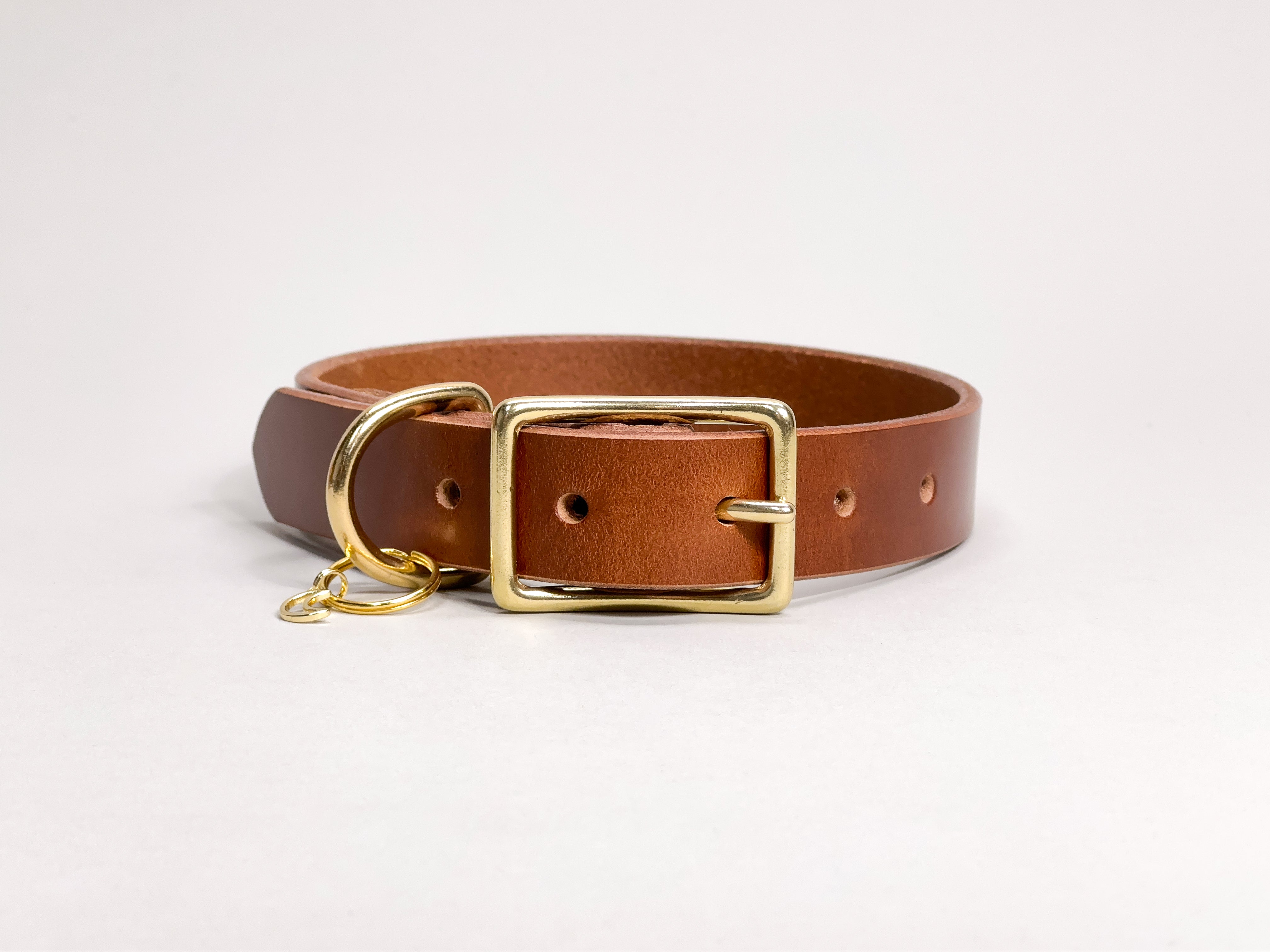This image features a brown leather belt coiled neatly on a plain, beige-colored background. The belt appears fairly wide, approximately one and a half inches, and it has a simple, straightforward design. You can observe that it's made from real leather, noticeable along its edges. Central to the belt's appearance is its rectangular gold buckle, currently fastened through the third of five equally spaced holes. Additionally, the belt includes a gold loop to secure the loose end and a small, circular gold keychain attached to it. Despite its size, the belt looks compact and finely crafted, possibly reminiscent of a dog collar due to the photo's perspective.